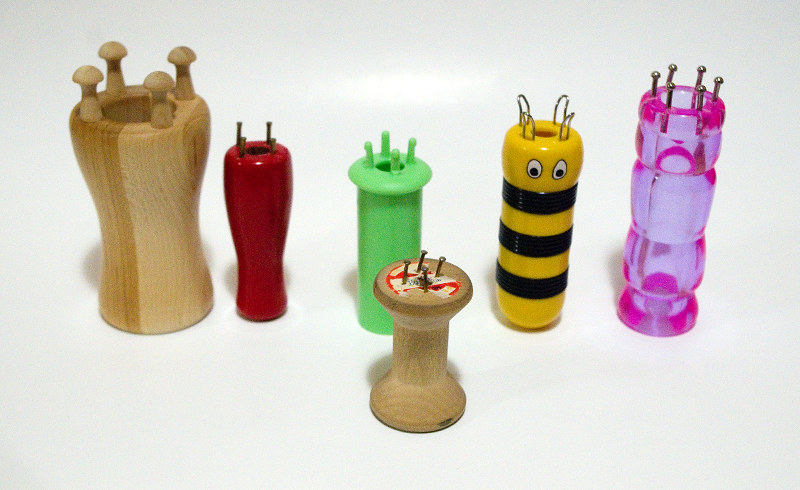This color landscape photograph, taken on a white tabletop, features six small cylindrical objects with equidistant pins or pegs protruding from the tops. Positioned on the table, the objects cast visible shadows, confirming the tabletop setting. The objects vary in material, with some being plastic and others wooden. Starting from the left, a large wooden piece with an inward curve resembling an hourglass is prominent. Next to it is a red plastic cylinder followed by a straight green one. A unique piece, decorated in yellow and black stripes to resemble a bee, complete with two eye-like details, adds a whimsical touch. There is also a transparent pink cylinder, and in front of these, a short wooden object shaped like a spool. The pegs or pins, ranging from four to six per object, suggest the items might be used for activities involving tying knots, braiding, or weaving, hinting at their possible functionality as crafting tools.